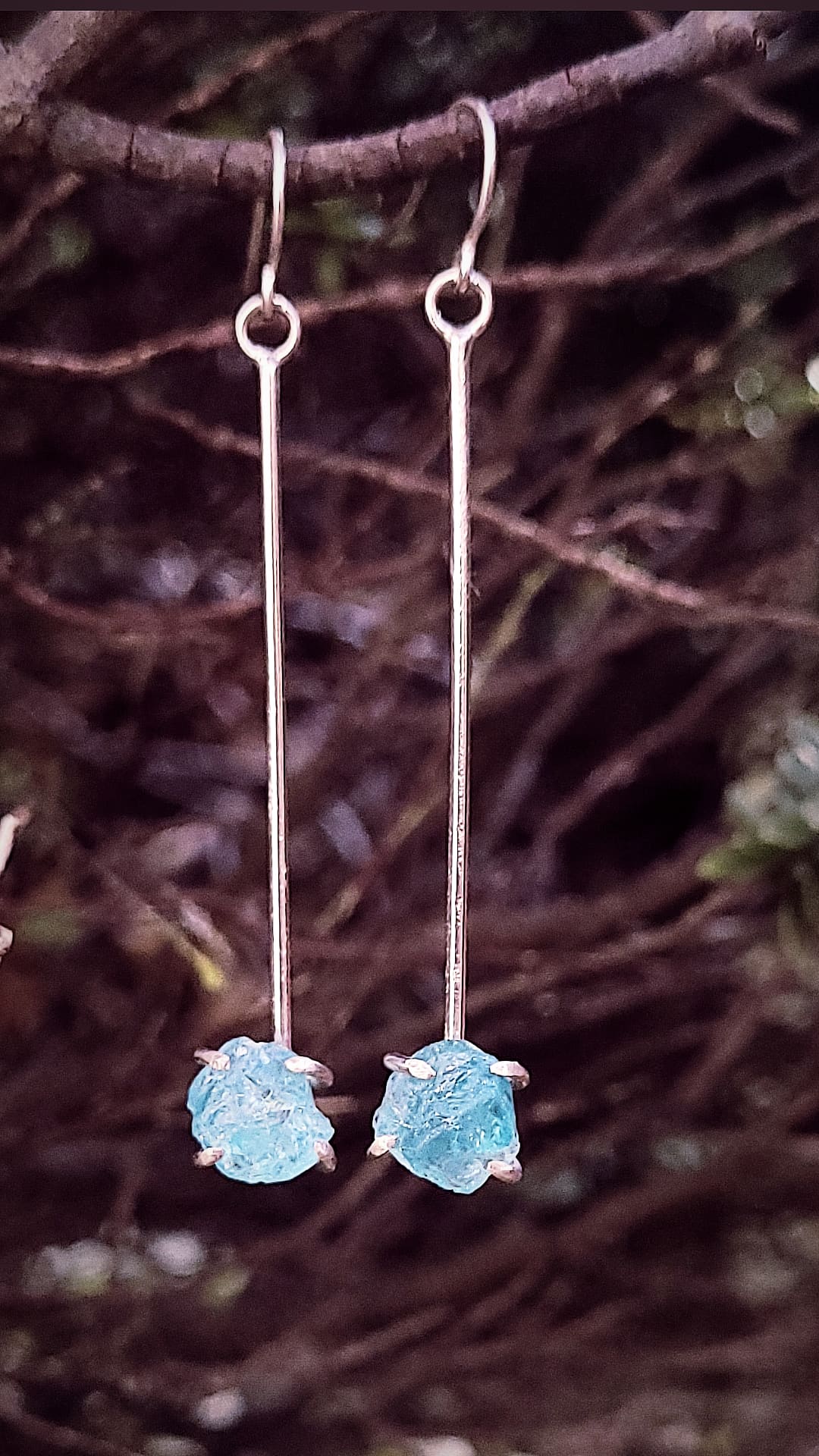The photograph showcases a rustic and detailed display of a pair of exquisite earrings. The main focal point is a close-up of a brown branch in the foreground, against a softly out-of-focus backdrop of piled twigs and branches. Lightweight, delicate flowers can be faintly discerned among the branches. A key branch stretches diagonally from the left to the right across the image, gracefully supporting the dangling jewelry. The earrings themselves feature long, silver stems with translucent, rough-cut blue gemstones, possibly aquamarines, held securely by intricate prongs. These stones, described as both blue rubies and aquamarines, exhibit a beautiful, almost ethereal quality that catches the light. The display gives off a natural, almost country-like ambiance, reminiscent of a scenic location, and effectively emphasizes the rustic elegance of the earrings, suitable for an artisanal marketplace listing.